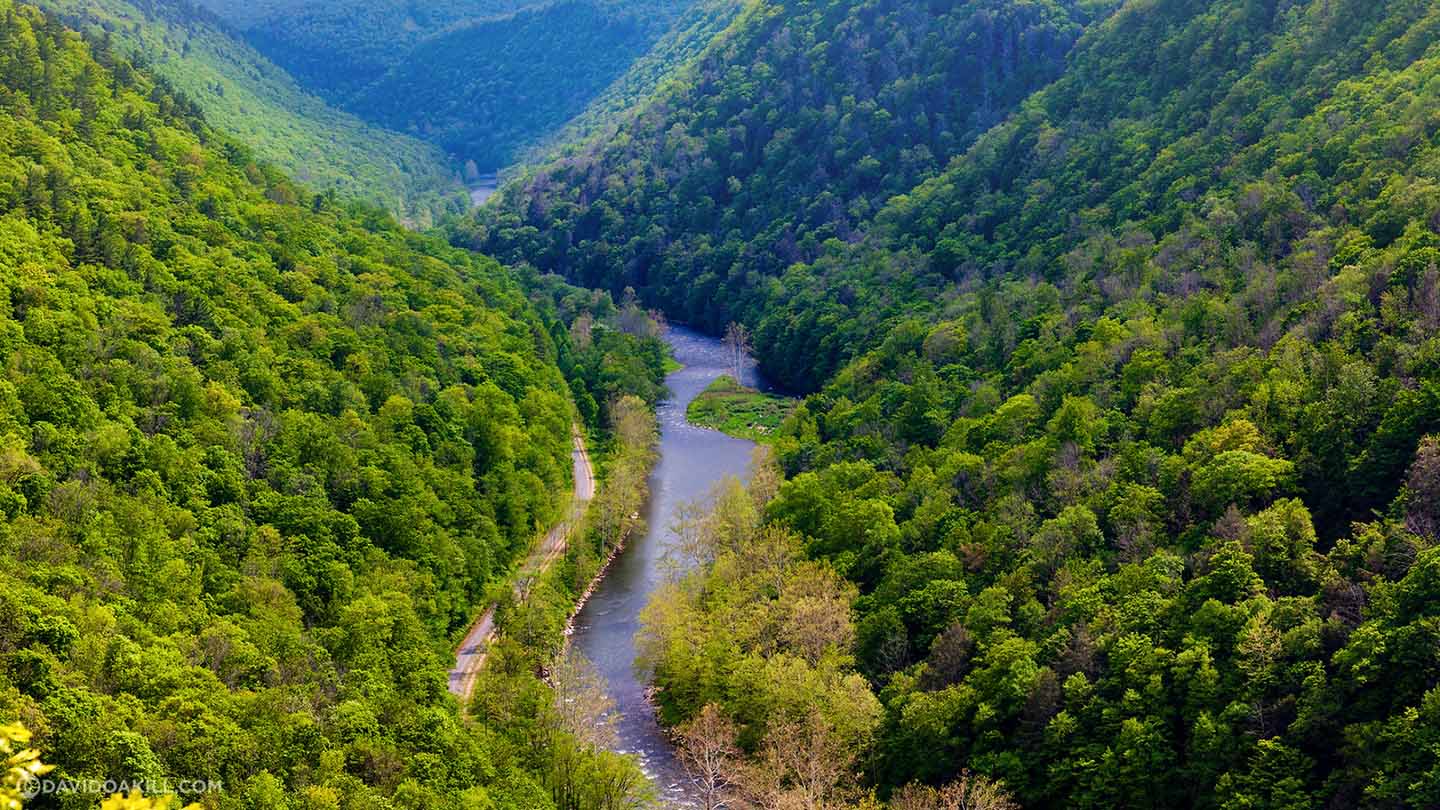This serene landscape photograph captures a winding, light blue river flowing through the heart of a lush valley. Taken from a high vantage point, the image offers a broad, zoomed-out view revealing an abundance of green foliage on both sides. The left side features a curved road lined with a dense mix of bright green trees, some showing hints of purple hues. Similarly, the right side is adorned with clusters of light green trees, interspersed with occasional patches of purple. The trees appear densely packed, masking the ground beneath, with a few exhibiting a light yellow or brown tint, suggesting a seasonal transition. The scene is devoid of human presence, buildings, or any indication of weather, painting a tranquil portrait of nature, possibly in late summer or early fall.